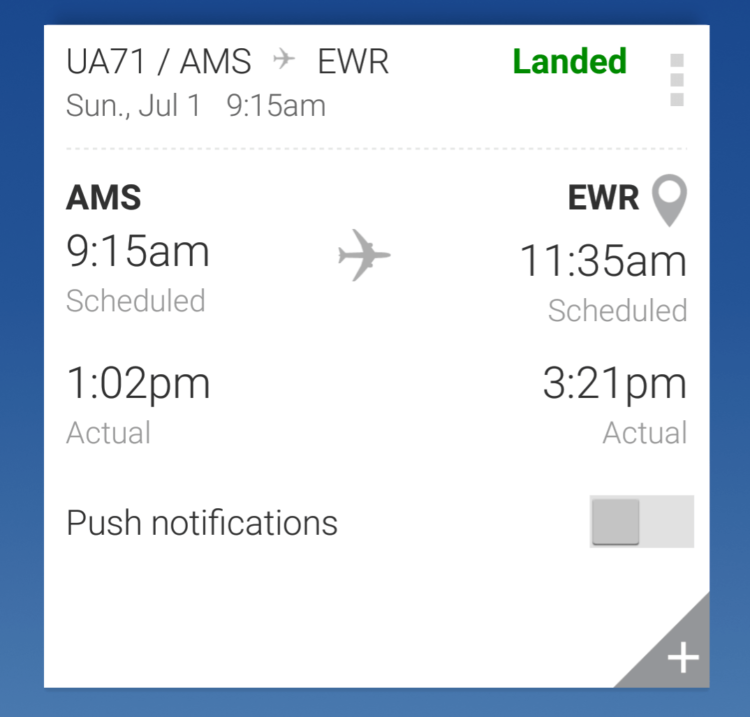The image depicts a portion of a smartphone screen displaying an airport app interface. The page is dedicated to flight information. At the top, it prominently features the flight code "UA71/AMS" in uppercase letters, alongside an airplane icon flying towards the right. Next to this text, "EWR" is also in uppercase.

To the right, in green text, the word "Landed" indicates the flight status. Below this information, there are three vertical squares. A dotted line separates additional flight details: 

- "AMS" in uppercase, signifying the Amsterdam airport.
- Below "AMS" is the scheduled landing time, "9:15 AM."
- An airplane icon in mid-flight is centered in this section.
- To the right, "EWR," the Newark airport, is indicated.
- Beneath "EWR" is the scheduled arrival time, "11:35 AM."

Further down, the actual landing times are specified:
- "1:02 PM" beneath "AMS."
- "3:21 PM" beneath "EWR."

Towards the bottom, there's a section mentioning push notifications, which are currently turned off. The bottom-right corner features a white addition symbol on a gray background. The entire interface is framed with a blue border, against a predominantly white background.